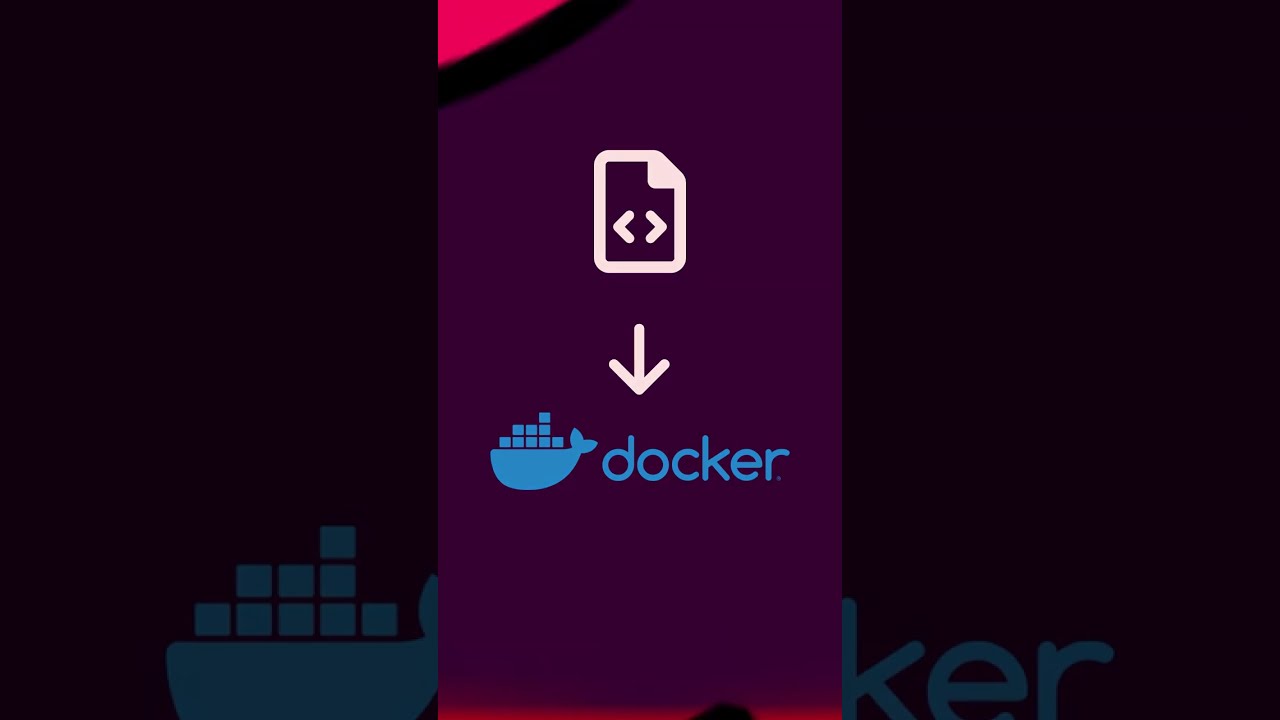The image is a screenshot resembling a social media post, possibly from TikTok or Instagram, featuring branded content for Docker. The central element is the Docker logo, which consists of a pale blue whale silhouette carrying ten small square blocks on its back. The word "Docker" is displayed in lowercase with a blue font adjacent to this whale icon. Above the Docker text is a white downward-pointing arrow, and further above is a white document icon. The background prominently features a deep purple or plum color scheme, with an enlarged and partially transparent Docker logo repeating in the backdrop. In the top left corner, a portion of a vivid red circle with a black outline is visible, adding a contrasting highlight to the composition.